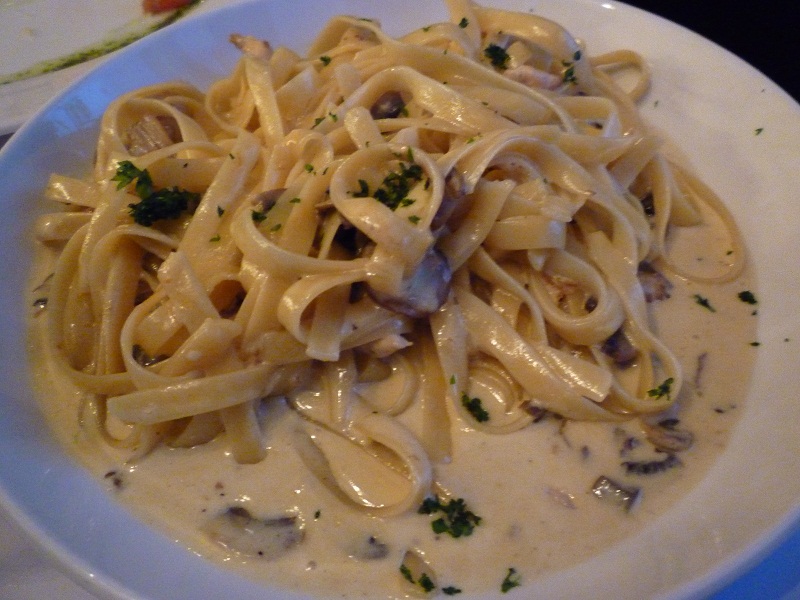This is a detailed photograph of a white, round glass plate filled with a generous serving of fettuccine Alfredo. The flat, cream-colored noodles are evenly coated in a rich, glossy Alfredo sauce, giving them a slightly yellowish hue. Interspersed among the pasta are vibrant green broccoli florets and sautéed brown mushroom slices, adding both color and texture to the dish. Fresh parsley is sprinkled on top, contributing a fragrant, herbal note to the composition. The plate rests on a dark table, with the table's edge subtly visible on the right side of the image. In the upper left corner, the edge of another plate with only a few crumbs is partially visible, suggesting this could be part of a larger dining setting. The sauce appears moderately ample, generously bathing the noodles, hinting at a creamy, hearty meal intended for one person.